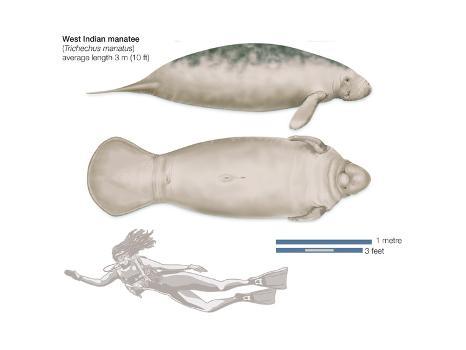The image is a detailed informational display in black and white focusing on the West Indian manatee. At the top, the title reads "West Indian manatee" in dark font. The display includes two stacked illustrations of a manatee, followed by a drawing of a diver girl. The first illustration at the top presents a profile view of a manatee, highlighting its gray mottled dark back, light gray side and bottom, small eyes, and two flippers, alongside a flattened tail. The second illustration beneath it depicts the manatee from an upside-down perspective, showcasing its pale underside. Below these manatee illustrations, there's a drawing of a girl wearing full scuba gear, complete with fins, a mask, and a vest, to provide a comparative scale for the animal's size. To the right of the images, there is a graph indicating one meter and three feet to help gauge the manatee's average length, which is noted to be around 10 feet.